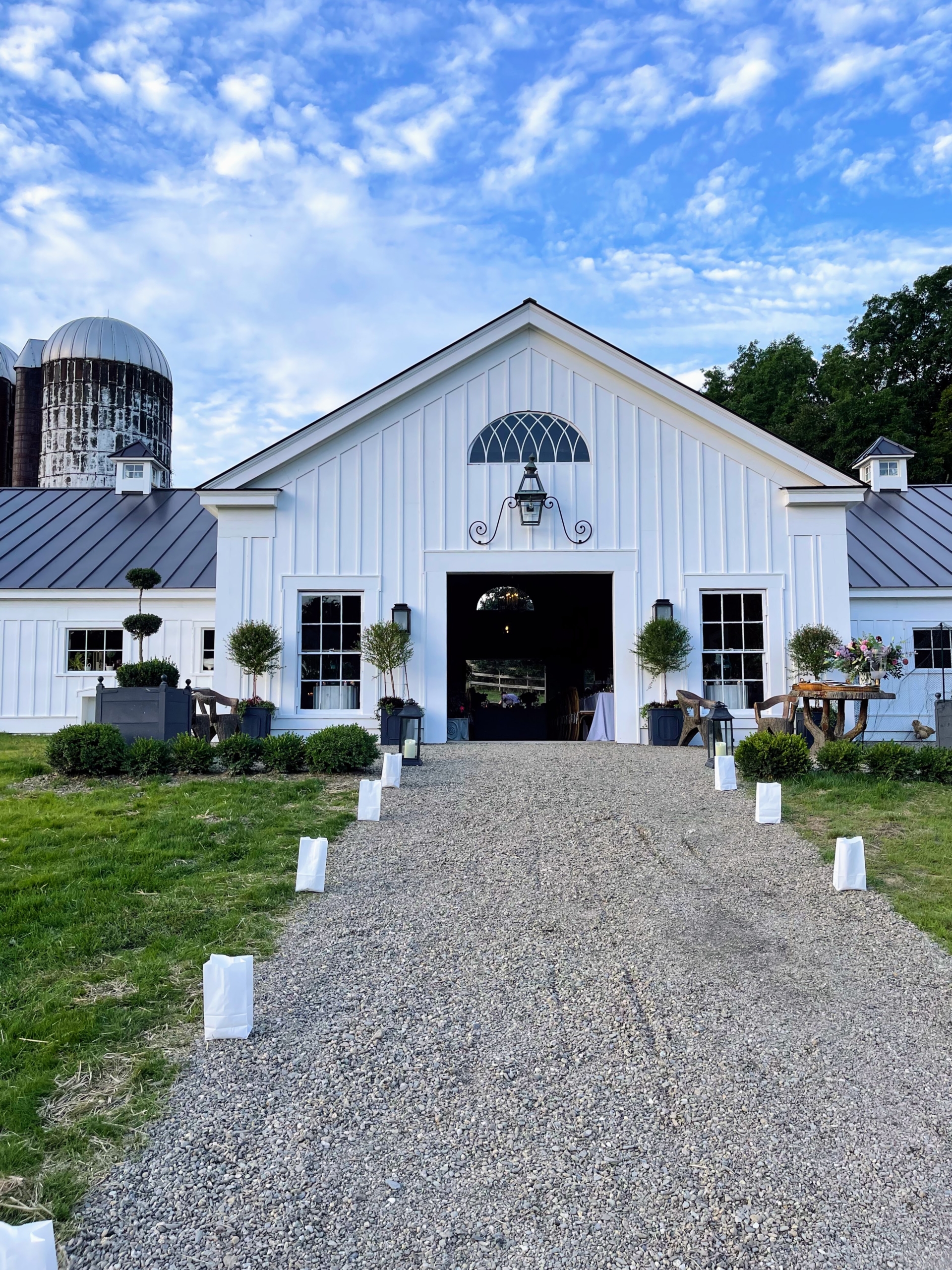The image depicts a small, white building, possibly a fancy barn or wedding venue, bathed in the serene light of a cloudy blue sky. The building is adorned with a black roof, showing signs of wear and peeling paint. The front door, centrally located and open, is framed by a gravel driveway that leads straight to the entrance. Flanking the doorway is a decorative, unlit lamp in a lantern casing, with elegant spiral lines extending from its sides. Directly above the lamp is a charming half-circle window featuring intricate plant-like floral curves, adding a rustic elegance to the facade. 

On either side of the door, there are multiple windows that enhance the building's inviting look. The right of the image reveals green trees and a black grain silo, which is weathered but adds to the picturesque farm-like setting. In front of the building, neat bushes line the façade, while a lush field of grass extends on both sides, occasionally dotted with hay. Adding to the outdoor charm, small lamp posts are positioned next to the windows, providing a quaint and welcoming atmosphere. The entire scene is enveloped in an ambiance that hints at it being a desirable location for rustic weddings and gatherings.